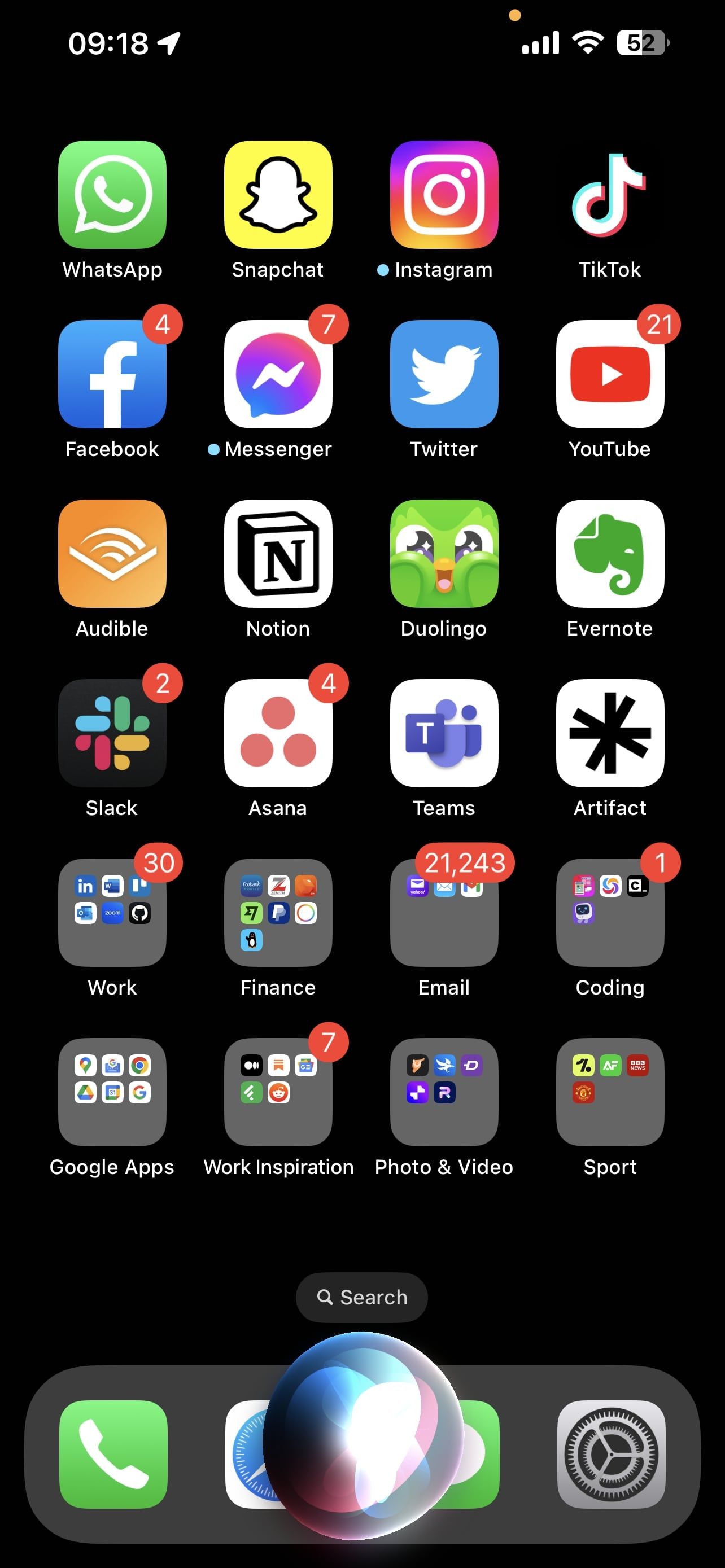Screenshot of an iPhone home screen taken at 9:18 AM, based on the clock displayed in the top left corner. The top right corner shows the signal strength, a Wi-Fi icon, and the battery percentage at 52%. 

The home screen features six rows of app icons arranged from left to right:
- **Row 1:** WhatsApp, Snapchat, Instagram, TikTok.
- **Row 2:** Facebook (4 notifications), Messenger (7 notifications), Twitter, YouTube (21 notifications).
- **Row 3:** Audible, Notion, Duolingo, Evernote.
- **Row 4:** Slack (2 notifications), Asana (4 notifications), Teams, Artifact.
- **Row 5:** Four category folders: "Work" (30 notifications), "Finance," "Email" (21,243 notifications), and "Coding" (1 notification).
- **Row 6:** Google Apps, Work & Inspiration (7 notifications), Photos & Video, Sport.

The bottom bar (dock) contains Phone, Safari, Messages, and Settings apps. Siri is activated, as indicated by the highlighted Siri icon on the screen.